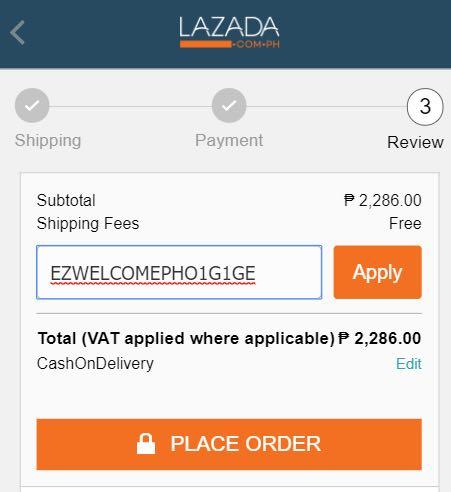The image depicts the final stages of the checkout process on Lazada.com.ph, a popular e-commerce platform. At the top of the image, the Lazada logo is prominently displayed in white text against a dark blue-teal gradient background. The logo features the word "LAZADA" in all capital letters with a unique design where the horizontal bar of the 'A' is a swooping arc rather than a flat line. Beneath the word "LAZADA," there is an orange bar and the URL "COM.PH" follows in a smaller font.

Below the logo, the checkout progress is illustrated through a series of three connected circles. The first circle, labeled "Shipping," is grey with a checkmark, indicating that the shipping details have been completed. A line connects this circle to the second circle in the middle of the screen, which is also grey with a checkmark and labeled "Payment." A final line leads to the third circle on the right side of the screen, numbered "3" and labeled "Review," signifying the current step in the checkout process.

The bottom half of the image focuses on payment information. It lists the order subtotal as ₱2,286.00, with a special currency symbol featuring three lines through it. Shipping fees are marked as "FREE," directly below the subtotal. There is a section for entering a promotional code, which displays the code "EASYWELCOME PH01G1GE" in all caps. To the right of this code is an orange "APPLY" button. Notably, the promo code text is underlined in red, suggesting a potential spelling or entry error.

The total amount remains consistent with the subtotal, and the payment method is specified as "Cash on Delivery" with an adjacent blue "EDIT" button for modifications. At the very bottom of the image, an orange "PLACE ORDER" button spans the width of the screen, featuring white text in all capital letters centered within the button, inviting the user to finalize their purchase.